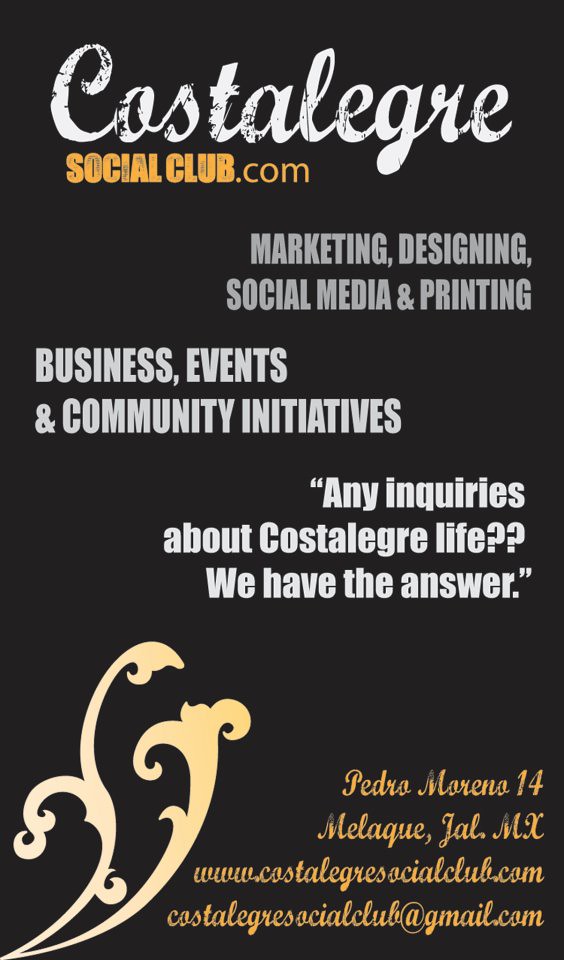The promotional poster features a sophisticated design with a solid black background. At the top of the poster in a white chalk-like font, it reads "CosTalagri." Below this, in bold yellow-orange letters, it states "SocialClubs.com." The center portion of the poster includes grey text listing the services, with "Marketing, Designing, Social Media, and Printing" on the right side, and "Business, Events, and Community Initiatives" on the left. A notable line of text on the right emphasizes, "Any inquiries about CosTalagri life, we have the answer." The poster’s bottom left corner showcases two abstract beige or pale yellow flower patterns with long stalks. In the bottom right, orange text provides the additional details: "Petra Marana, 14, Malacute, JAL MX," followed by the website "www.CosTalagriSocialClub.com." This promotional piece effectively combines illustration, graphic design, and typography to create an eye-catching and informative advertisement.